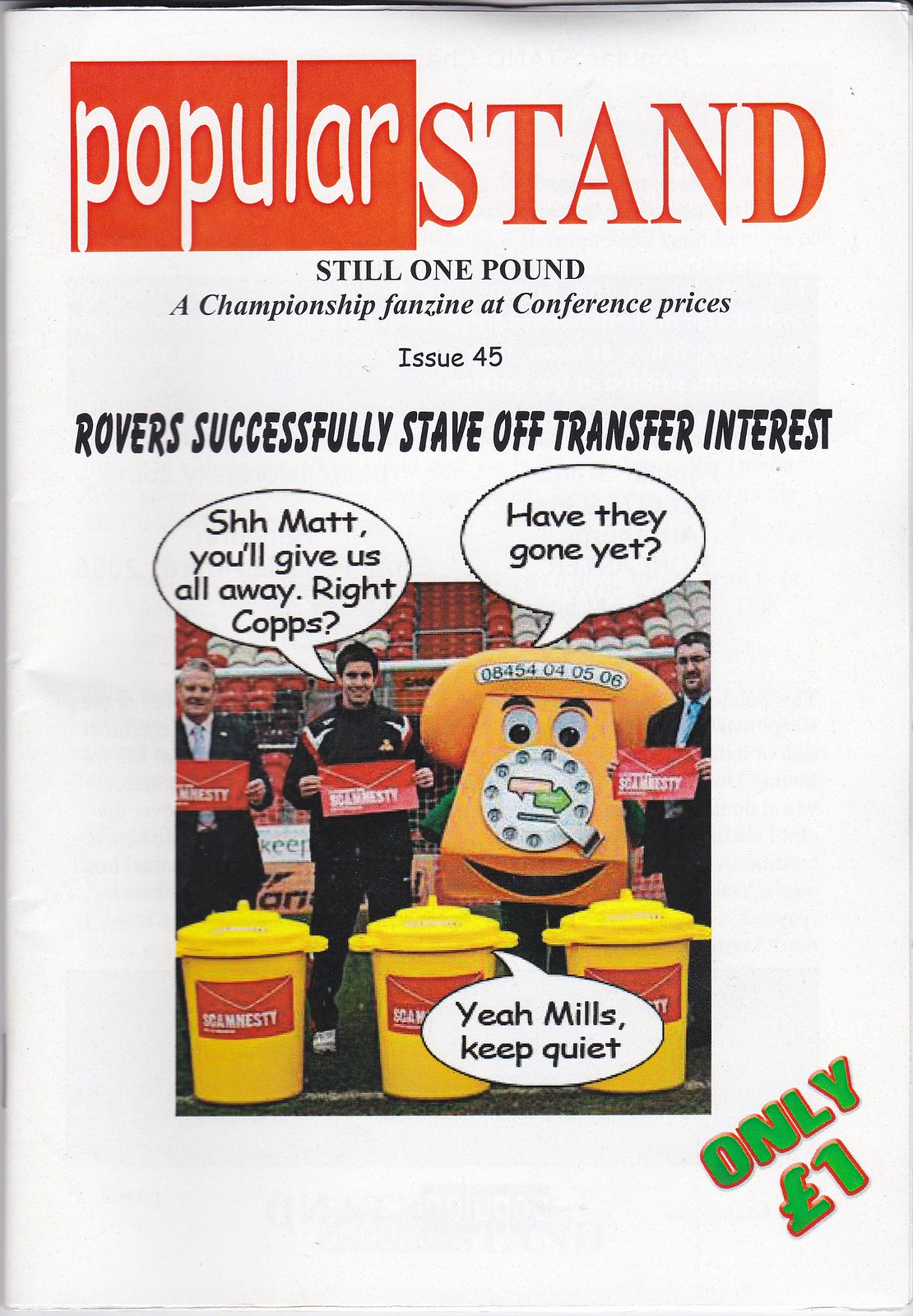The image is of the cover of a magazine called "Popular Stand," with the subtitle "Still One Pound" and the tagline "A Championship Fanzine at Conference Prices." This particular issue is number 45, featuring the top story, "Rovers Successfully Stave Off Transfer Interest." The central visual element is a cartoon-like illustration with conversation bubbles. The illustration features two men and a mascot designed as an orange rotary telephone with a person's legs visible underneath. One man is wearing a suit, and the other is in a warm-up tracksuit. They are positioned in front of three large yellow receptacles that resemble either trash cans or oversized cups. The man in the tracksuit says, "Shh, Matt, you'll give us all away, right, cops?" while the telephone mascot asks, "Have they gone yet?" A voice from one of the yellow receptacles adds, "Yeah, Mills, keep quiet." In the bottom right corner, there is green text stating, "Only One Pound."